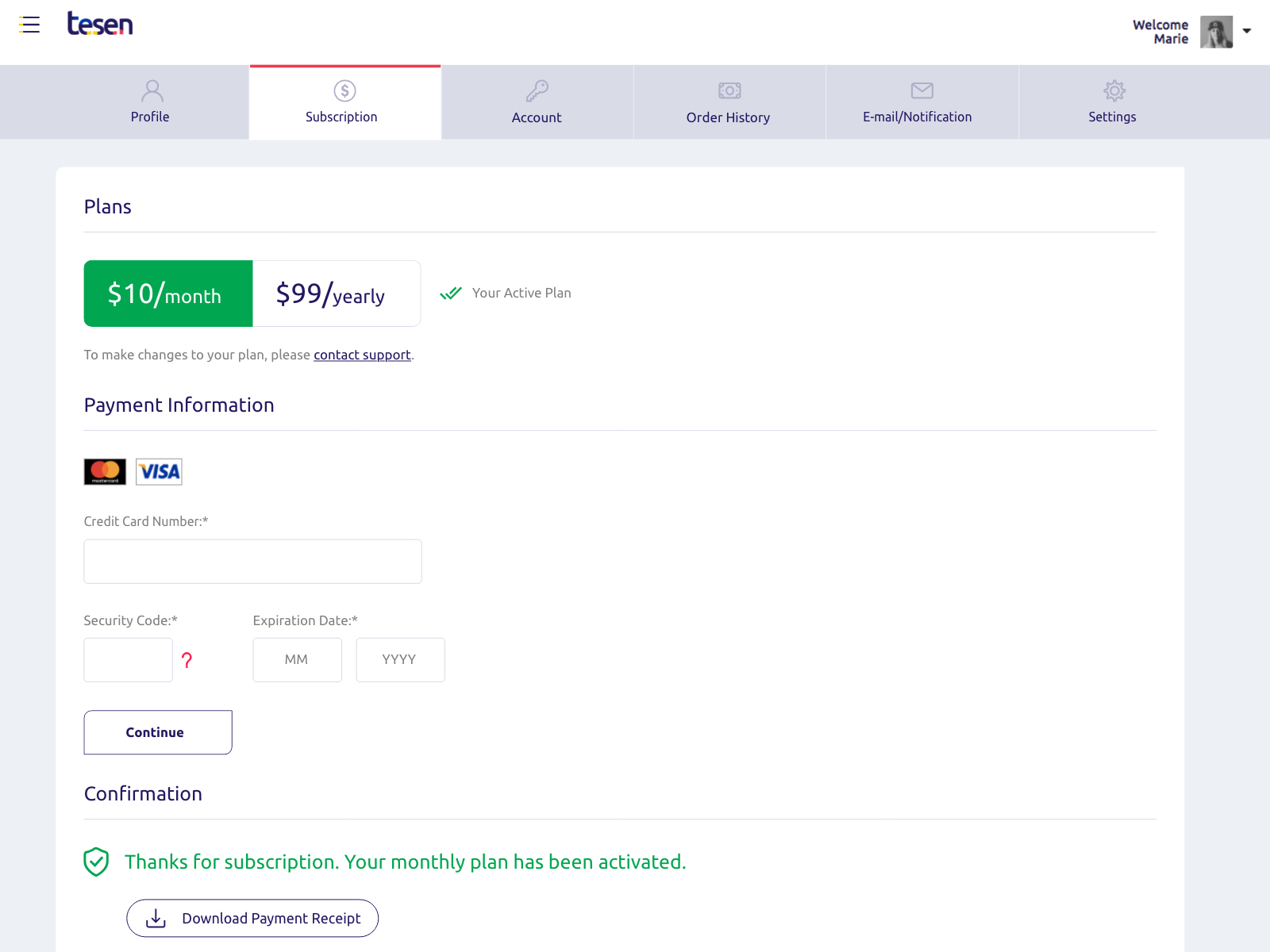This image is a screenshot of a subscription management page on a website called TESEN. The interface features a white background with a light gray border and a medium gray header bar. At the top of the page, in the upper left corner, the brand name "TESEN" is prominently displayed. On the right-hand side of the header, there is a black and white profile picture with a dropdown menu labeled "Welcome Marie."

The navigation menu on the left includes six headings: Profile, Subscription, Account, Order History, Email/Notification, and Settings. The "Subscription" tab is currently selected and highlighted in white.

The main content area under the subscription tab displays a section titled "Plans." Here, users can choose between a $10 per month plan or a $99 yearly plan. The $10 per month option is currently selected, marked by a green highlight. A note below this section instructs users to contact support for any changes to their plan.

Further down, the page shows payment information fields with icons for MasterCard and Visa. Users are required to enter their credit card number, security code, and select the card’s expiration month and year from dropdown boxes. A blue "Continue" button is available for proceeding with the payment.

At the bottom of the page, a confirmation message is displayed with a green-bordered check mark, stating "Thanks for your subscription. Your monthly plan has been activated." Along with this, there is a thin button featuring an arrow icon labeled "Download Payment Receipt" for users to obtain their payment confirmation details.